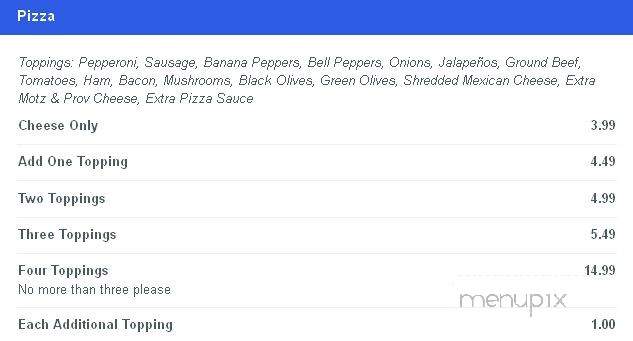The image is a screenshot of a pizza menu. At the top of the image, a prominent blue bar displays the word "Pizza" in white font on the top left. Below the blue bar, there is a blank white space followed by some text in italics. Beneath the italicized text, the list of available toppings is displayed, including pepperoni, sausage, banana peppers, bell peppers, onions, jalapeños, ground beef, tomatoes, ham, bacon, mushrooms, black olives, green olives, shredded Mexican cheese, extra mozzarella, provolone cheese, and extra pizza sauce.

To the right of the toppings list, there is a price chart specifying the cost of different pizza options. The prices are: 
- Cheese Only: $3.99
- Add One Topping: $4.49
- Two Toppings: $4.99
- Three Toppings: $5.49
- Four Toppings: $14.99 

Additionally, a note at the bottom of the list advises, "No more than three toppings, please," and mentions that each additional topping costs an extra $1.

At the bottom of the image, there's a watermark in light gray font that reads "menu PIX."